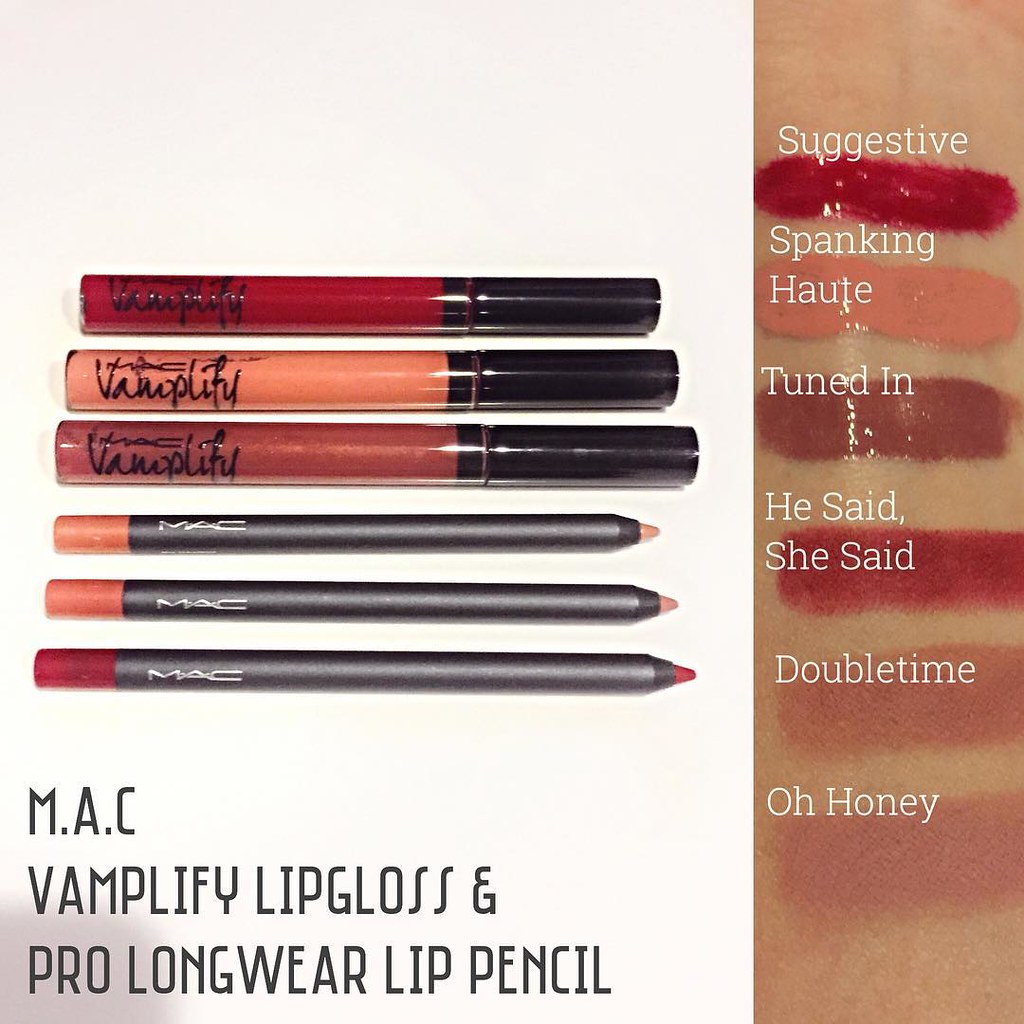This advertisement features a clean, white background on the left two-thirds, showcasing six makeup items—three lip glosses and three lip pencils—arranged horizontally. The lip glosses are capped and range in color from a dark reddish-pink to a peach and a lighter pink. Below these are corresponding lip pencils, also aligned horizontally, with the tips matching the gloss shades: peach, pink, and darker pink. Both product lines are from the same brand as indicated by the gray text below them that reads, "MAC Vamplify Lip Gloss and Pro Longwear Lip Pencil."

The right one-third of the image contrasts with a pink background and features a vertical strip displaying swatches of the makeup on a skin-tone backdrop, demonstrating the colors' effects when applied. Labels over corresponding swatches read: "Suggestive," "Spanking Haute," "Tuned In," "He Said, She Said," "Double Time," and "Oh Honey," covering a spectrum from reddish-pink to peach and light pink. This provides a clear visual of how these products look on different skin tones, emphasizing their variety and application.